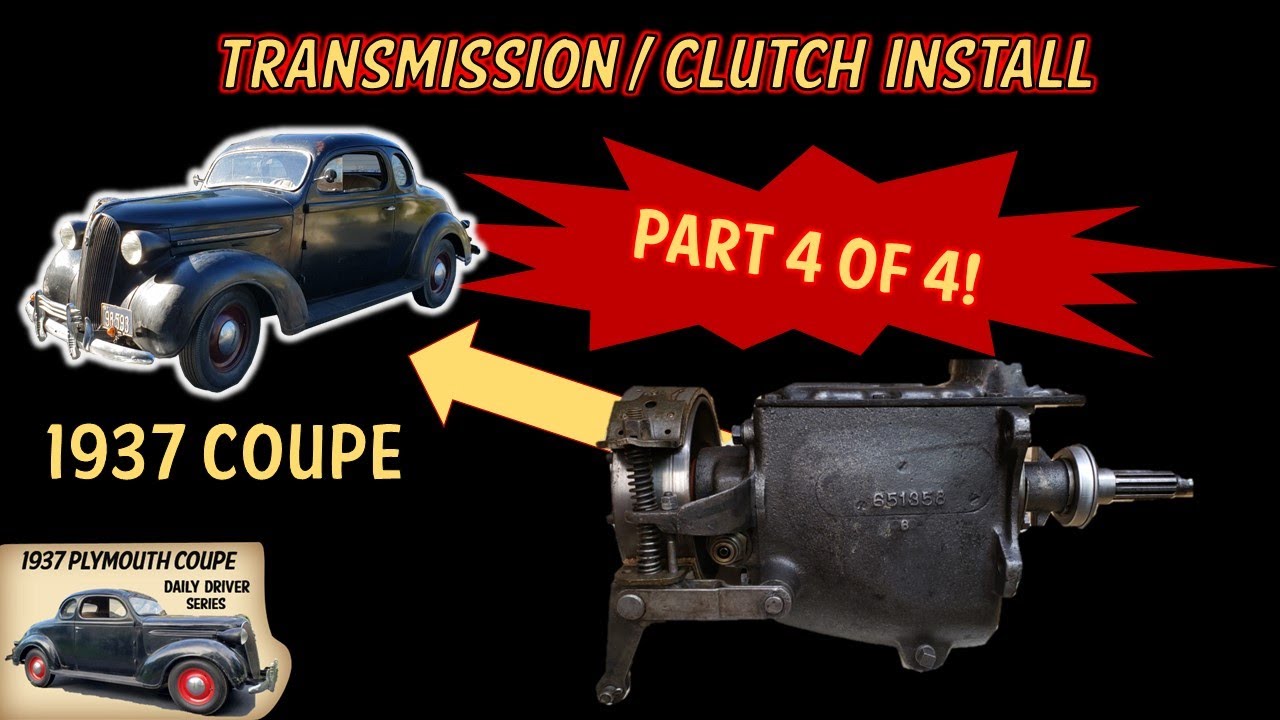The landscape-oriented image, set against a black background, prominently features an old-fashioned, black two-door 1937 Coupe with black wheels and a white outline, situated on the left side. Above the car, bold yellow text outlined in red reads "TRANSMISSION / CLUTCH INSTALL" in all caps. To the right of the car, there is a red splatter with yellow text at its center that says "PART FOUR OF FOUR!" in uppercase letters. Below the car, in yellow text against a black background, is the label "1937 COUPE." Adjacent to this label, on the right side, is a black and silver engine profile, which has a bold yellow arrow diagonally pointing from the engine to the car, indicating their connection. The image altogether resembles an illustrative splash screen or thumbnail for a video.